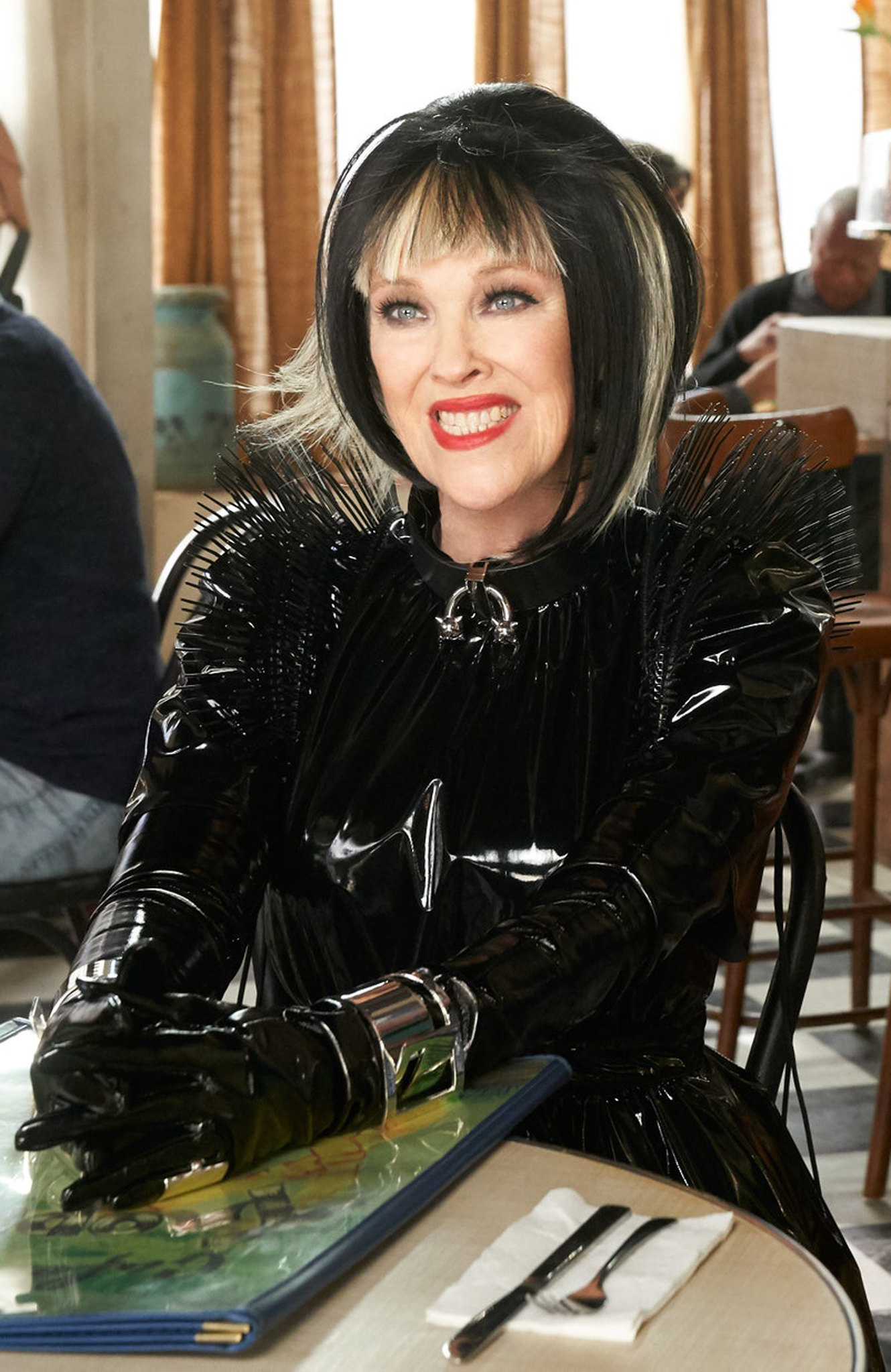In the photograph, a woman is seated at a round wooden table in a restaurant, with her hands resting over a blue menu. She is the focal point of the image, smiling brightly with visible teeth and adorned with striking red lipstick. Her skin is fair, and she has meticulously styled black hair interspersed with blonde highlights, fashioned into short bangs and an asymmetrical bob. Her bright blue eyes and well-manicured eyelashes add to her captivating appearance. 

She is dressed in a distinctive, black, leather-like uniform resembling a goth style, complete with spikes around the shoulders and matching black gloves. A silver bracelet, or possible sharia, encircles her wrist. The table in front of her also holds a white napkin, a knife, and a fork. 

In the background, brown curtains hang against the wall, and other diners are seated at various tables, adding to the lively ambiance of the restaurant. The woman sits on a black chair, fully engaged in the moment, emanating a vibrant and compelling presence that dominates the scene.